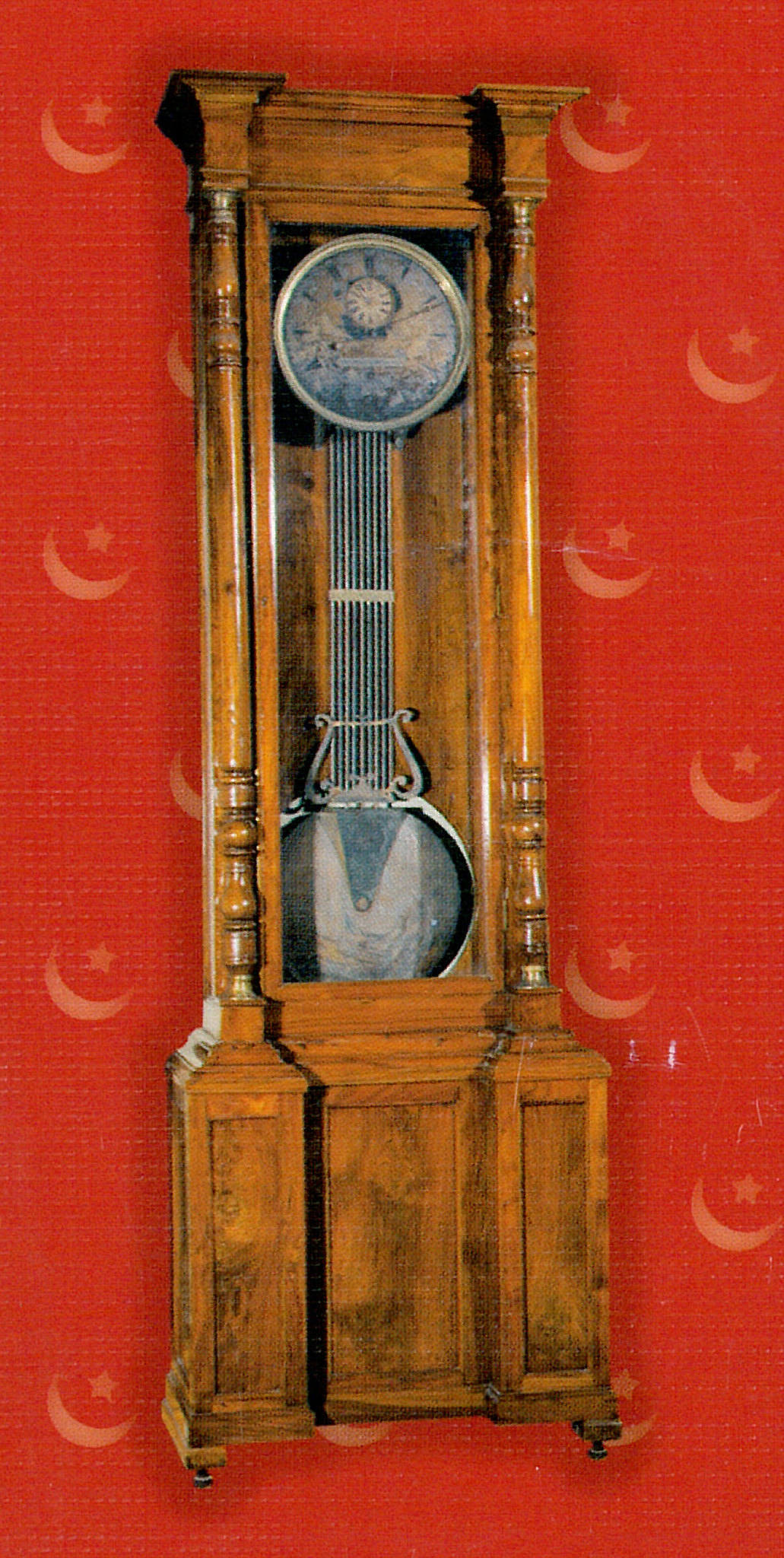The image features a beautifully aged grandfather clock, exuding an antique charm. The clock is encased in what appears to be varnished wood, giving it a rich, warm appearance with hues of cherry, light browns, dark browns, and blacks. The decorative wooden frame encases a glass door, allowing a view of the clock's intricate internals. The face plate of the clock, positioned at the top, displays an unusual and intriguing design, adorned with shades of blue, teal, black, and white. 

The lower portion of the clock showcases a pendulum, adding to its classic elegance. The clock stands on four black pegs, each accented with a ring of white, elevating the base slightly above the ground. In the background, there is a striking red backdrop featuring a crescent moon and a star, further enhancing the clock's vintage allure. This detailed image captures the timeless beauty and intricate details of the grandfather clock, making it a captivating piece of history.